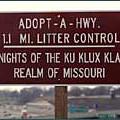The image is a small square photograph depicting a brown street sign with white lettering, mounted on a rectangular wooden post. The sign contains four lines of text, starting with "Adopt-A-Highway" and "1.1 Mi Litter Control," followed by "Knights of the Ku Klux Klan," and "Realm of Missouri." The background reveals a suburban or small-town setting, including a mix of trees and grass, with distant buildings—one white and one brown—visible beyond the sign. The image also includes elements such as a few people, green street signs, and a brick building far in the background, suggesting the sign might be captured from a higher vantage point looking over a cityscape or town. The photograph itself is roughly an inch and a half square in dimension.